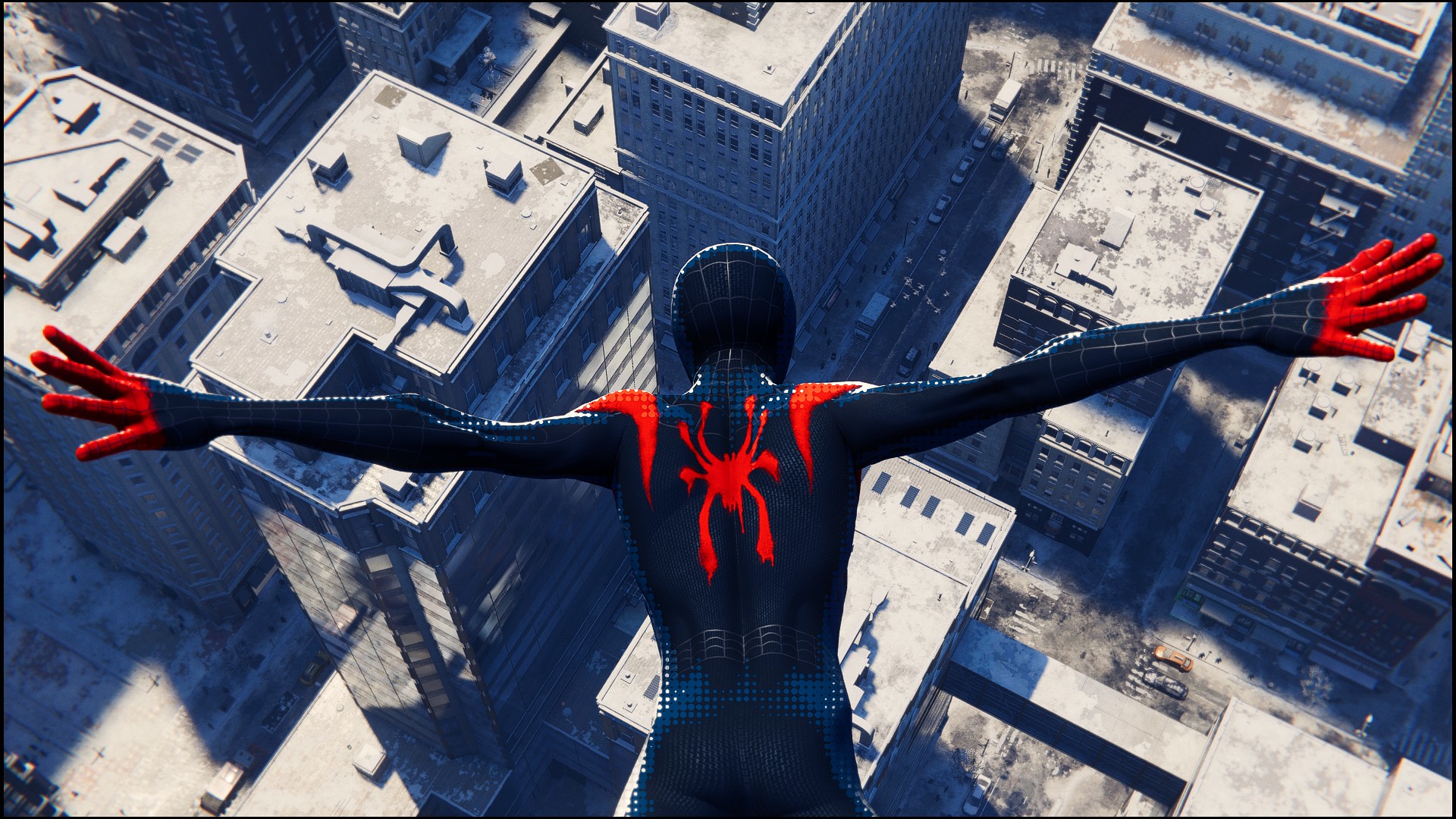The image is a dynamic aerial view, either a photograph or a stylized photorealistic drawing, capturing a superhero clad in a dark blue bodysuit embellished with intricate spiderweb patterns. The figure, resembling Spider-Man, has his back to the viewer, arms outstretched as if in mid-fall or flight. The suit features striking red accents: a red eight-legged spider emblem on the back, red shoulders, and red gloves extending from just below the fingertips. The hero's head is covered by a matching blue hood. Below, a sprawling cityscape unfolds with gray high-rises, their rooftops bathed in sunlight casting sharp shadows. The streets are visible with minuscule cars and trucks navigating the traffic, with a parking lot filled with parked cars in the lower right quadrant. The sun's rays highlight parts of the buildings, creating a striking contrast between illuminated and shadowed areas, adding depth to the urban environment.